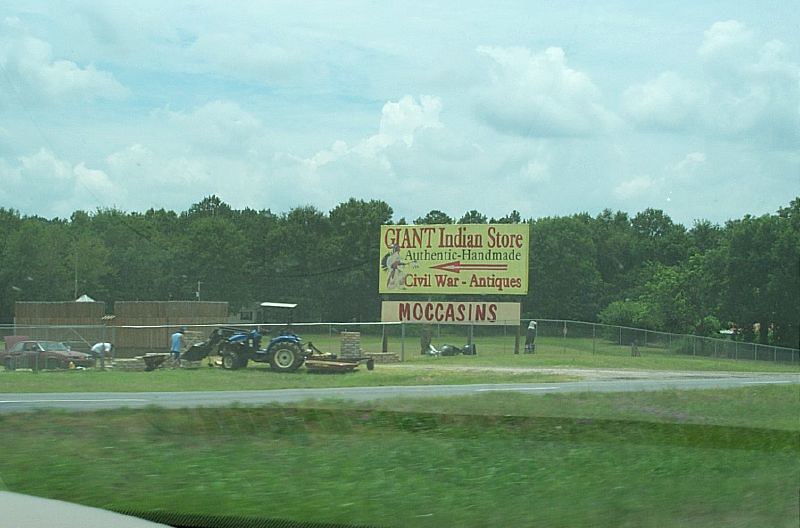The image depicts a rural business area dominated by a large yellow billboard that reads, "Giant Indian Store - Authentic Handmade Civil War Antiques," beneath which is a sign that says "Moccasins." The billboard features a red arrow pointing left, guiding visitors toward the store. The scene is set against a backdrop of tall trees lining the perimeter of the lot, framing a clear blue sky with fluffy white clouds.

The foreground consists of an overgrown green field and a small chain link fence running along it. A blue tractor with a trailer is positioned near the gate, with two men working nearby; one in a blue tank top at the front of the tractor and another in a white shirt bending over. Additionally, a brown compact car is parked close to them. 

In the background, a structure made of wood is under construction, indicating ongoing development on the property. The entire scene exudes a sense of rural enterprise, with the large trees providing a natural border and enhancing the secluded ambiance of the area.